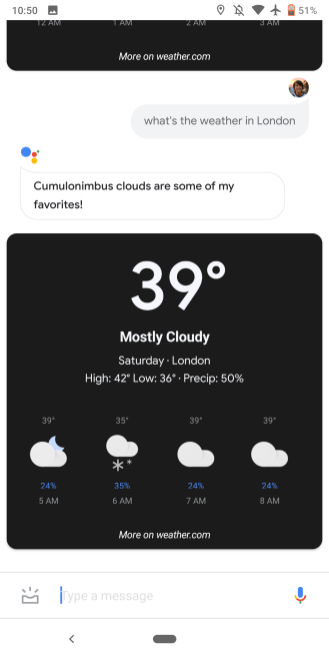A detailed smartphone screenshot depicts the current weather conditions via a weather application. At the top-left corner, the time reads 10:50. Adjacent to it is a small, indistinguishable icon. The far-right corner displays five different icons: a location services icon, a crossed-out notification bell indicating notifications are off, a Wi-Fi signal icon, airplane mode, and a red battery indicator signifying low battery.

Directly beneath, a black banner with a white font displays “Move on weather.com.” To the right, there is a small circular icon showing a person’s image, presumably the user’s profile picture. Below this, a chat interaction is visible. The user has queried, “What’s the weather in London?”

The response from what appears to be an AI chat assistant shows three colorful circles (blue, yellow, and orange) and begins with text indicating a personal touch: "Clouds are some of my favorites." The lower section of the screen, against a black background with white text, provides detailed weather information: "39 degrees, mostly cloudy, Saturday, London, high 42, low 36, precipitation 50%." A graphical representation of different times of the day shows icons for clouds, sun, and moon, reflecting varying weather conditions.

At the bottom of the screen, another search field is present, equipped with a microphone icon on the right, allowing users to input queries via voice command.